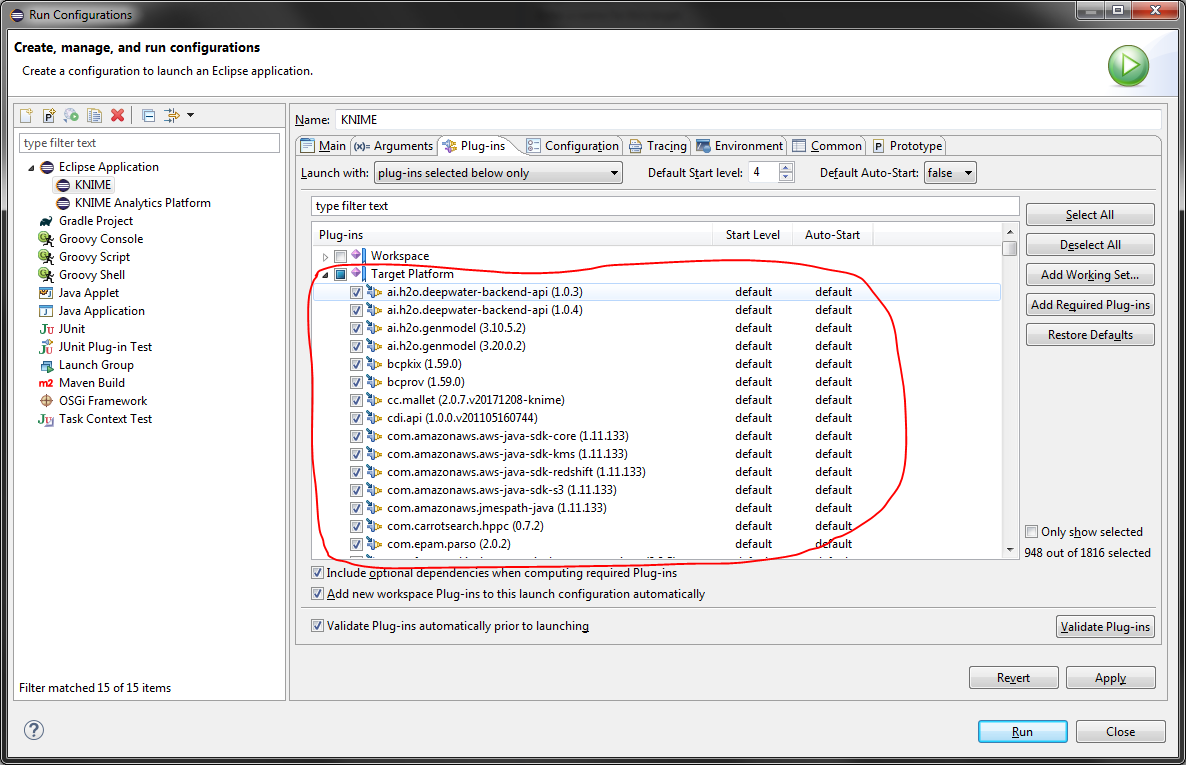A detailed screenshot of a computer screen displaying the "Run Configurations" window in an Eclipse IDE environment. At the top left, it prominently displays "Run Configurations" with a subtitle in black on white reading "Create, Manage, and Run Configurations." Below this, it further instructs, "Create a configuration to launch an Eclipse application." The main section to the left lists various configuration options, including "Gradle Project," "Groovy Console," "Groovy Script," "Groovy Shell," "Java Applet," "Java Application," down to "Task Context Test."

To the right, the central pane features the address bar, stating "Launch with Plugins Selected Below Only." A red circle outlines items such as "Workspace" and "Target Platform," along with a list of coded entries starting with "com.epam.parso," appended with "(20-2)." Columns labeled "Start Level" and "Auto Start" consistently display "Default." In the lower right corner, the options "Validate Plugins," "Revert," "Apply," "Run," and "Close" are visible, with "Run" highlighted by a green triangle play button, indicating it might be or has been pressed. Overall, this detailed image captures the setup for creating, managing, and running various configurations within Eclipse, emphasizing the screen's various functionalities and options.